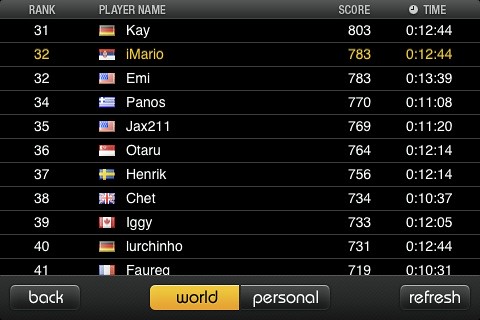The image depicts a detailed leaderboard for an unspecified sport, showcasing the rankings, player names, flags representing their countries, scores, and completion times. The board is predominantly black with white lettering, except for Rank 32, which is highlighted in yellow.

- **Rank 31**: K from Germany – Score: 803, Time: 12:44
- **Rank 32**: Amero (Unrecognized flag) – Score: 783, Time: 12:44 (Highlighted in yellow)
- **Rank 32 (Tie)**: EMI from the USA – Score: 783, Time: 13:39
- **Rank 34**: Panos – Score: 770, Time: 11:08
- **Rank 35**: Jax from the USA – Score: 769, Time: 11:20
- **Rank 36**: Arturo (Unrecognized flag) – Score: 764, Time: 12:14
- **Rank 37**: Henrik from Finland – Score: 756, Time: 12:14
- **Rank 38**: Chet from the UK – Score: 734, Time: 10:37
- **Rank 39**: Iggy from Canada – Score: 733, Time: 12:05
- **Rank 40**: Lurchino from Germany – Score: 731, Time: 12:44
- **Rank 41**: Farika from France – Score: 719, Time: 10:31

At the bottom of the screen are buttons for navigation, including a "Back" button, a "World" button highlighted in gold, a "Personal" button in dark, and a "Refresh" button in the lower right-hand corner.